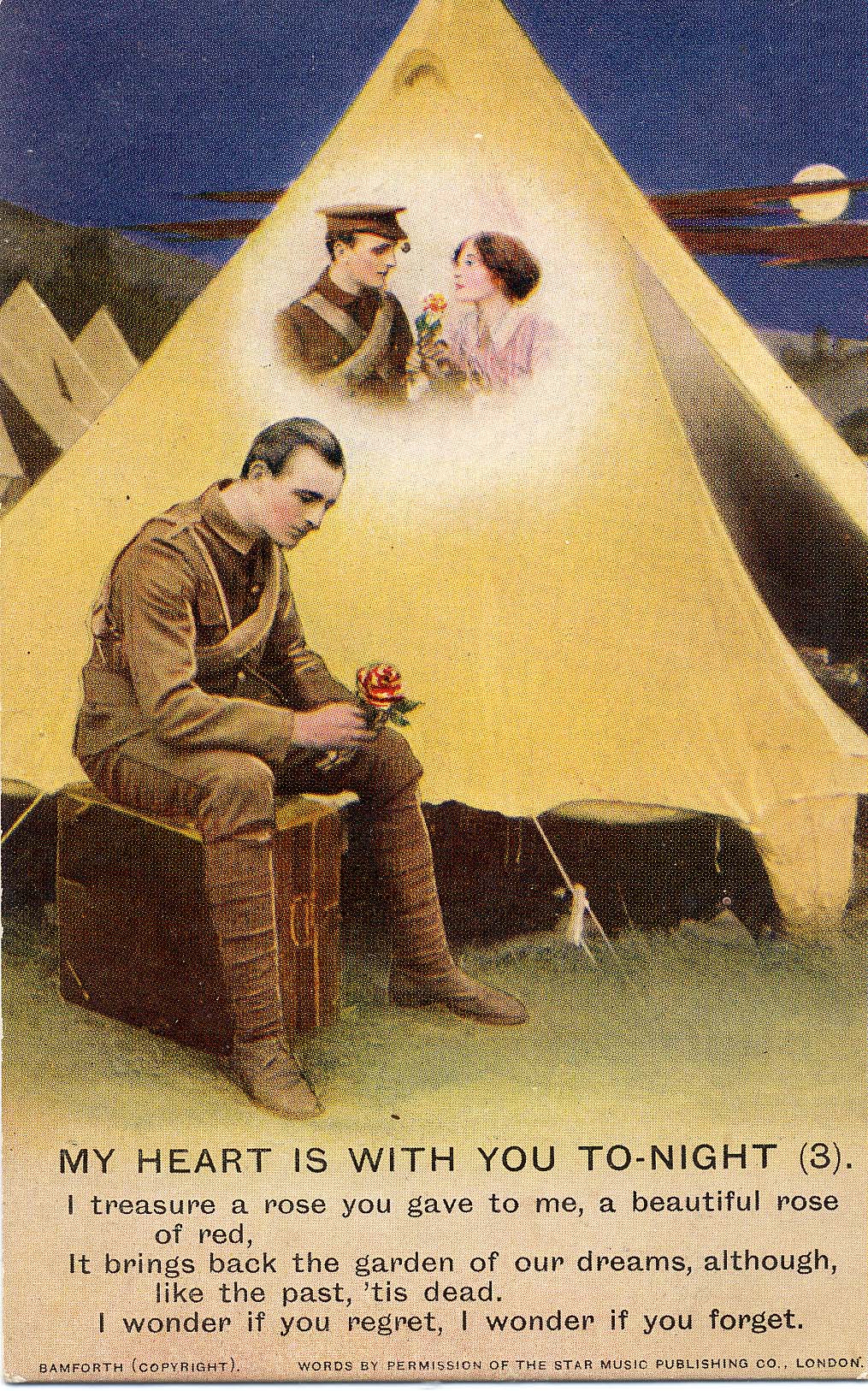In this evocative image, a forlorn soldier dressed in a brown military uniform sits on a suitcase before an open white tent set against the backdrop of a night sky adorned with the moon and clouds. The soldier, a white male with dark, slicked-back hair, gazes sadly at a red rose in his hand. Above him, projected onto a tent flap, is a nostalgic image of the same soldier wearing his cap and looking tenderly at a smiling woman of Caucasian descent who holds flowers, symbolizing his distant love. The image seems to be a print on canvas, possibly a page out of a book or magazine. Along the bottom of the picture, in black letters, is an inscription that reads: "My heart is with you tonight (3). I treasure a rose you gave to me, a beautiful rose of red. It brings back the garden of our dreams, although like the past it is dead. I wonder if you regret. I wonder if you forget." In the lower corners, the credits read, "Sam Forth Copyright" and "Words by permission of the Star Music Publishing Company, London." The poignant scene is rendered in tones of brown, yellow, and blue.